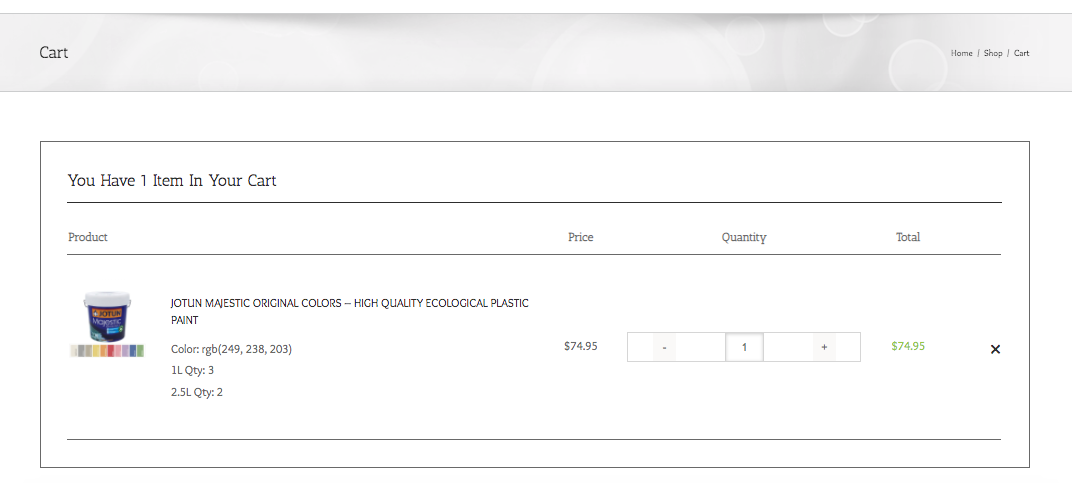The image portrays an online shopping cart interface. At the top left, the word "Cart" is displayed, highlighted by a subtle gray line. On the top right, small text options read "Home," "Shop," and "Cart." Beneath these, a message states, "You have one item in your cart."

In the main section, the product description reads: "Ioton, Majestic, Original Colors, High Quality, Ecological, Plastic Paint," accompanied by an image of a paint bucket to the left. Below the bucket, colorful stripes showcase the paint's available shades.

To the right, the product price is listed as $74.95, with a quantity of one. Adjacent to the quantity, plus and minus signs allow for quantity adjustments. The total cost reflects $74.95, and an 'X' symbol is positioned to the right for item removal.